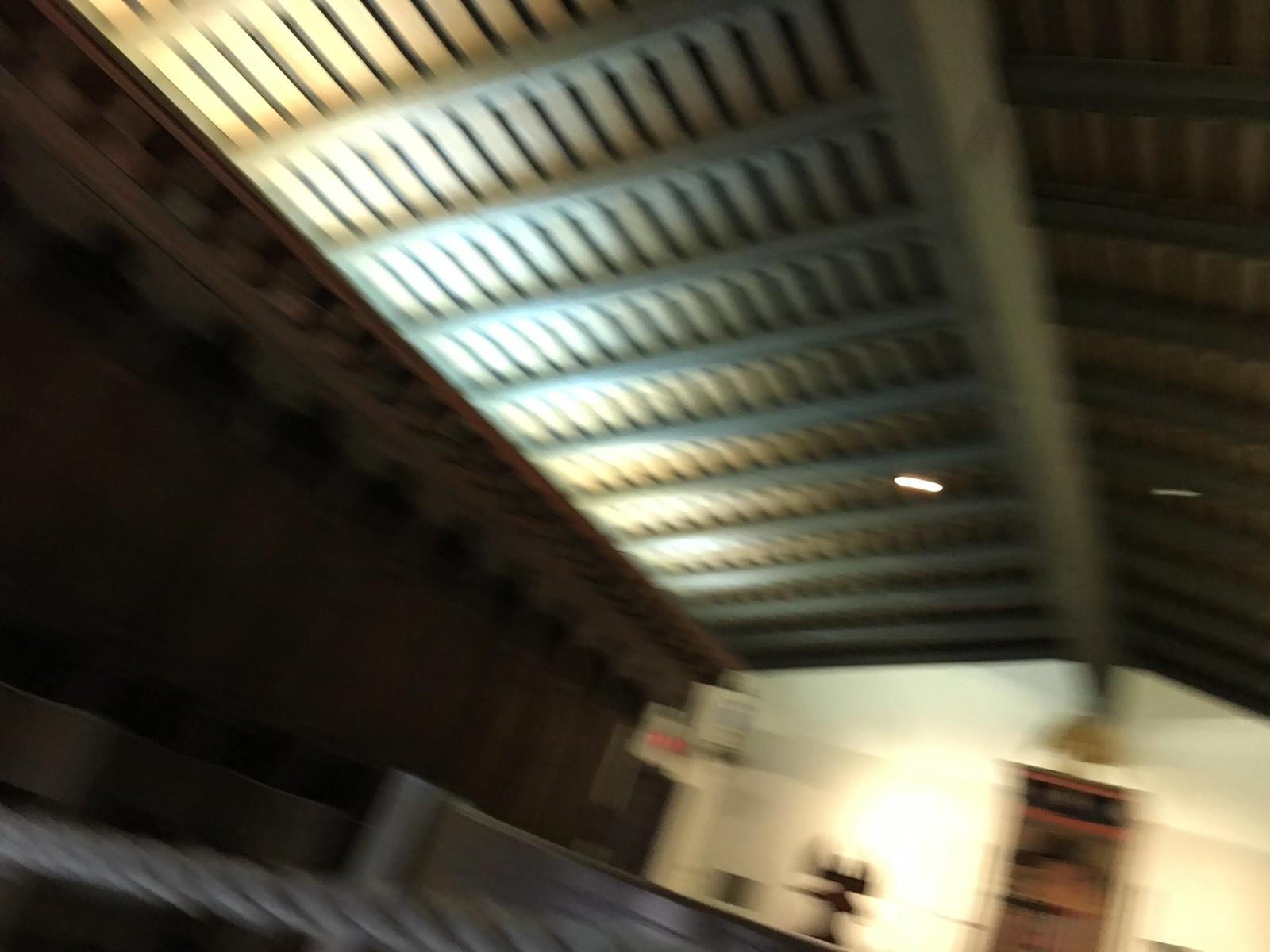The image depicts a wide, panoramic view of the interior of a structure, possibly a church. The photo is blurry, suggesting it was taken in motion or improperly rendered. The central focus is the roof, characterized by a series of white beams that converge to form a gentle A-frame, supported by a long rafter extending towards what could be the altar. Positioned on the wall, near the altar area, is a rectangular object, and to the left, there appears to be a sculpture. The left side of the image shows a visible wall and what seem to be pews at the bottom, though their details are obscured by the motion blur. The roof also features lighting elements, including a prominent light fixture and recessed lighting along the left side, illuminating the area where the congregation would typically sit.